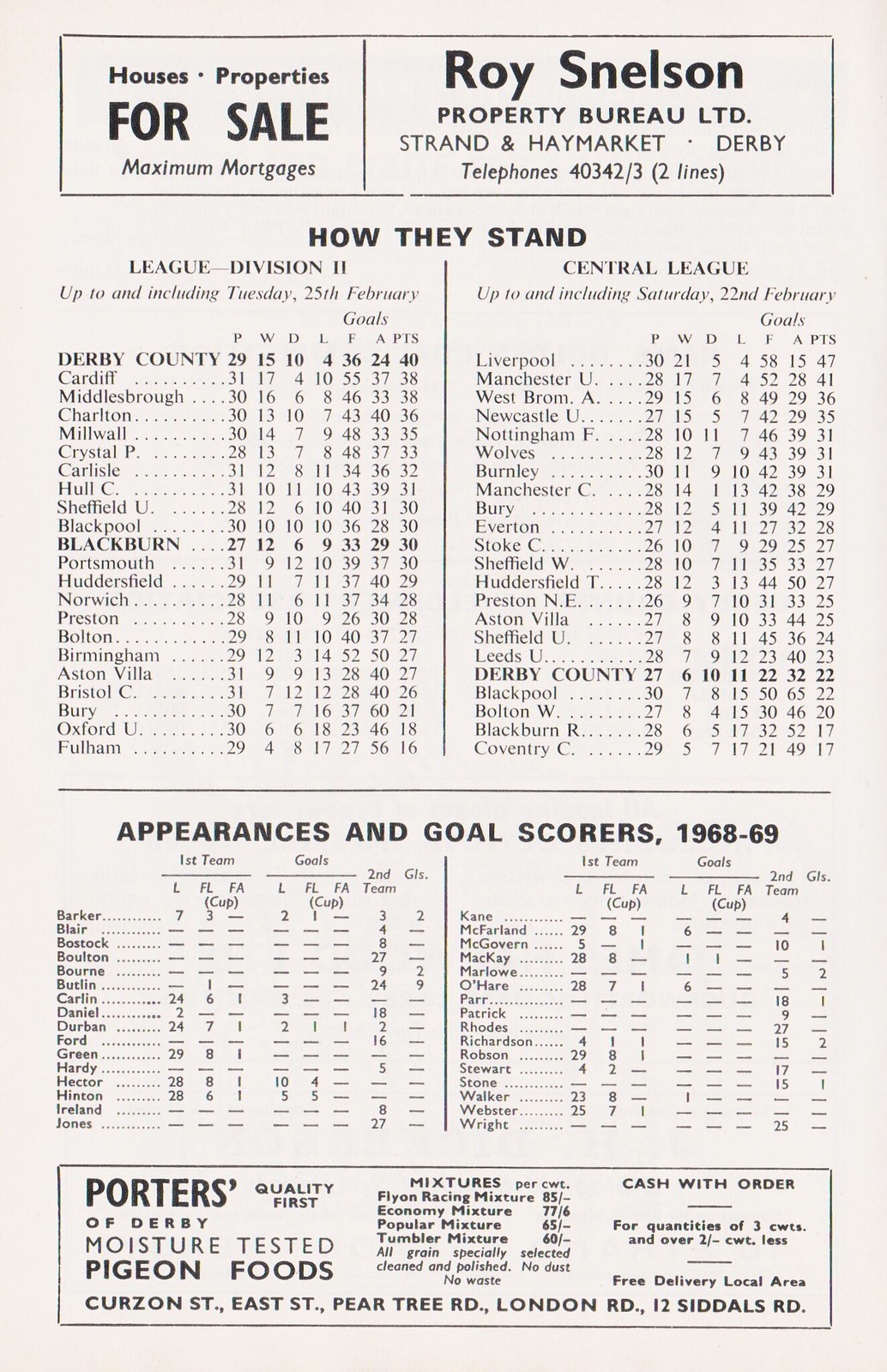The image captures a rectangular page, likely from a sports magazine or a stadium program, featuring detailed information and advertisements related to sports leagues. At the top, there's a prominent rectangular advertisement divided into two sections: the left section promoting "Houses, Properties for Sale, Maximum Mortgages" and the right showcasing "Roy Snelson Property Bureau Limited" along with its location at Strand and Haymarket, Derby, and a telephone number for contact. Below this, a title "How They Stand" introduces a chart categorizing and listing teams from "League Division 2" on the left and "Central League" on the right, detailing team standings with names like Derby County, Cardiff, Middlesbrough, Charlton, Millwall, and Crystal Palace. Further down, another set of charts titled "Appearances and Goal Scorers 1968 to 1969" meticulously provides player statistics, again divided into two sections. At the bottom of the page sits another rectangular advertisement for "Porters of Derby Moisture-Tested Pigeon Foods," detailing various mixtures and noting "Cash with Order" along with contact information for the business. The entire page is printed in black text on white paper, with small, precise lettering.